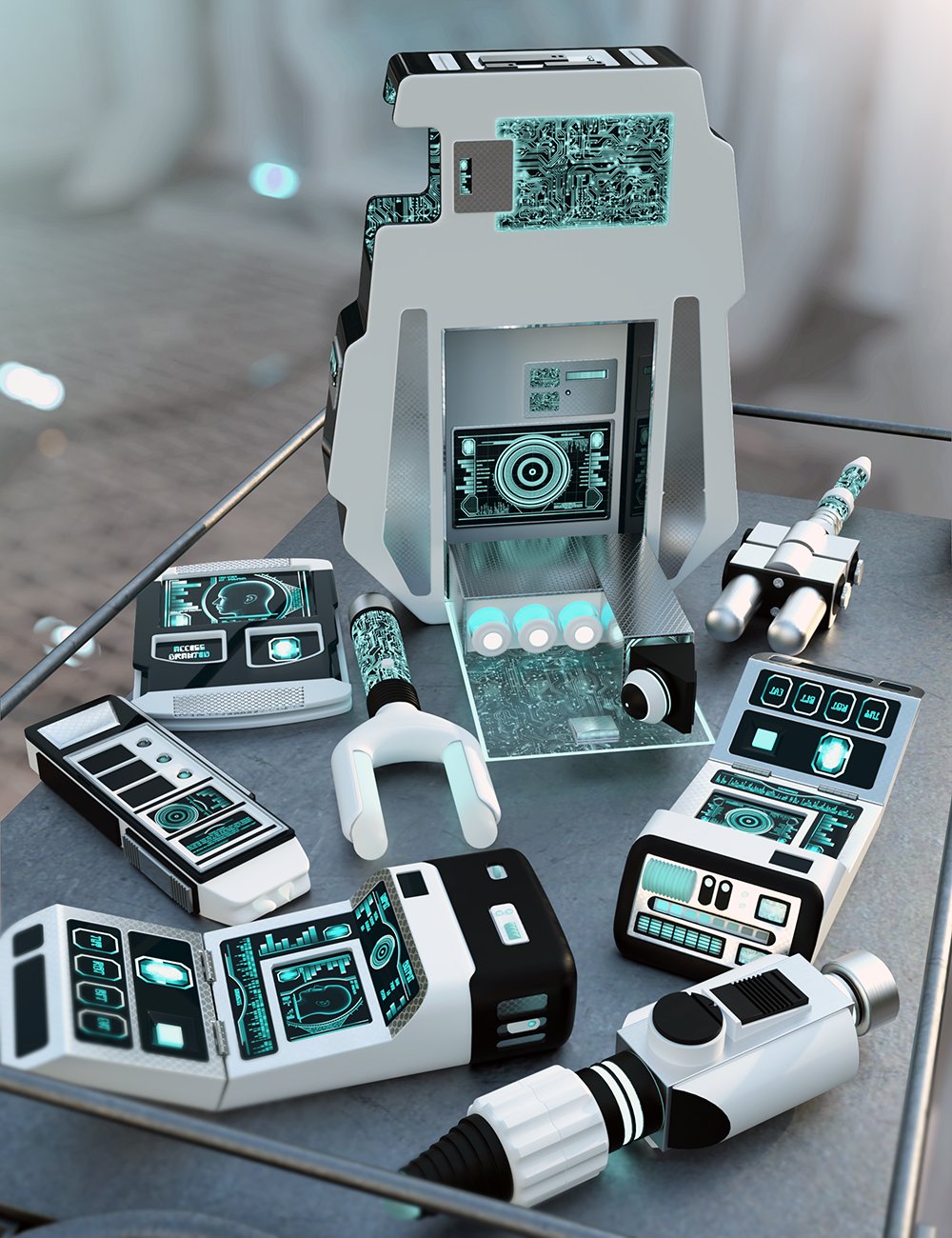This image depicts a collection of futuristic scientific tools arranged on a dark grey metal cart. The tools, possibly props for a movie, evoke a sci-fi aesthetic reminiscent of Star Trek. There are eight devices in total, each featuring a combination of white, black, and luminescent aqua blue colors. These gadgets are designed with various buttons, knobs, displays, handles, and other intricate components, presenting a sophisticated and advanced look. The largest tool is positioned in the corner, standing tall with a rectangular shape and notches along its side, adorned with a barcode or QR code at the top. The background is blurred, displaying only muted tones of grey, which further emphasizes the vibrant and intricate details of the tools on the cart.